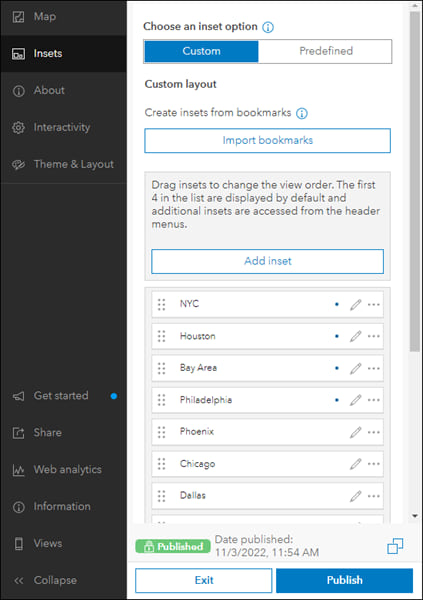This vertically styled page features a left sidebar with a sequence of interactive tabs. At the top, the tabs read "Map," followed by "Insets," "About," "Interactivity," and "Theme and Layout." Beneath these tabs is a gray spacer, and below it are additional navigable options: "Get Started," "Share," "Web Analytics," "Information," "Views," and "Collapse."

On the right side of the page, a section titled "Choose an Insert Option" is visible. Within this section, there are options for "Custom" and "Predefined," with "Custom" currently selected. This selection reveals more options: "Custom Layout," "Create Insets from Bookmarks," and a button labeled "Import Bookmarks."

Further down the page, users are instructed to "Drag insets to change the view order," with an explanation that the first four listed insets are displayed by default, and additional insets can be accessed from the header menus. There is also an "Add Inset" button for adding new insets.

Below this, a series of movable and editable boxes are displayed, labeled "NYC," "Houston," "Bay Area," "Philadelphia," "Phoenix," "Chicago," and "Dallas." 

At the bottom of the page, it notes that this content was published on November 3, 2022, at 11:54 a.m. Additionally, there is an "Exit" button and a prominently displayed blue "Publish" button.